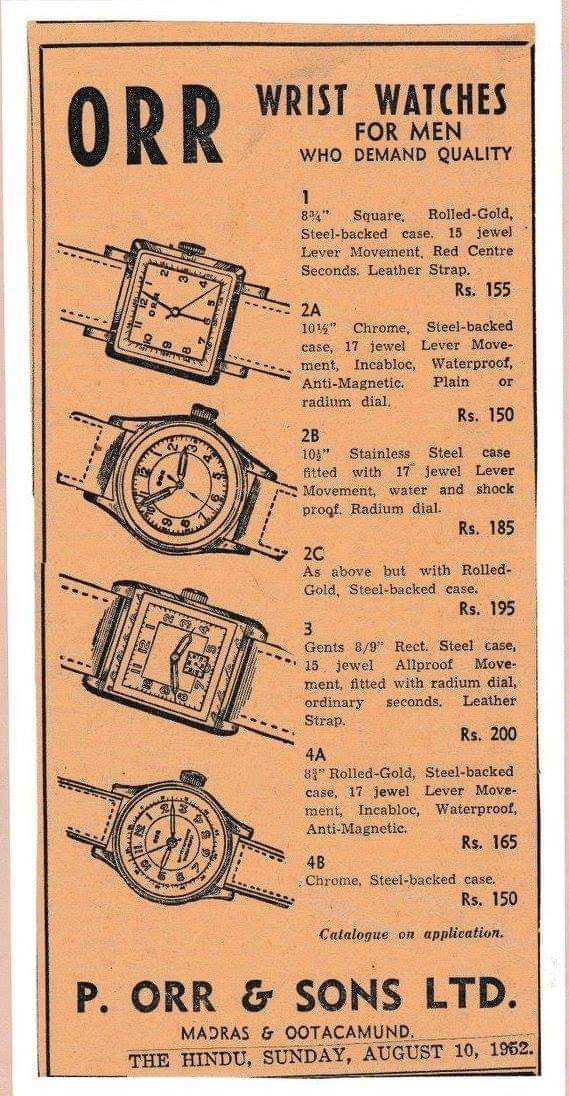This advertisement, likely clipped from an old newspaper or magazine dated August 10, 1962, features ORR wristwatches for men who demand quality. Set against a yellow or orange background with a black border, the ad displays black text and illustrations. The headline at the top reads "ORR Wristwatches for Men Who Demand Quality." On the left side, there are four detailed illustrations of watches—two are square-faced and two are round-faced. 

The right side provides detailed descriptions of seven different watch models, labeled 1, 2A, 2B, 2C, 3, 4A, and 4B. Model 1 features an 8¾-inch square, rolled gold, steel-backed case with a 15-jewel lever movement, red center seconds, and a leather strap, priced at RS155. Model 2A has a 10½-inch chrome, steel-backed case with a 17-jewel lever movement, ink block, waterproof, anti-magnetic features, and a plain or radium dial, priced at RS150. Model 2B is a 10½-inch stainless steel case with a 17-jewel lever movement, water and shockproof, and a radium dial, priced at RS185. Model 2C is similar to 2B but with a rolled gold, steel-backed case, priced at RS195. Model 3 is a gent’s 8/9-inch rectangular steel case with a 15-jewel, all-proof movement and radium dial, priced at RS200. Model 4A has an 8¾-inch rolled gold, steel-backed case with a 17-jewel lever movement, ink block, waterproof, and anti-magnetic features, priced at RS165. Model 4B is a chrome, steel-backed case, priced at RS150.

At the very bottom of the ad, the text states "Catalog on application" followed by the contact information "P.O.R and Sons Limited, Madras and Uttakamund," and specifies the source as "The Hindu Sunday, August 10, 1962." The detailed descriptions and visual illustrations emphasize the quality and variety of wristwatches available.